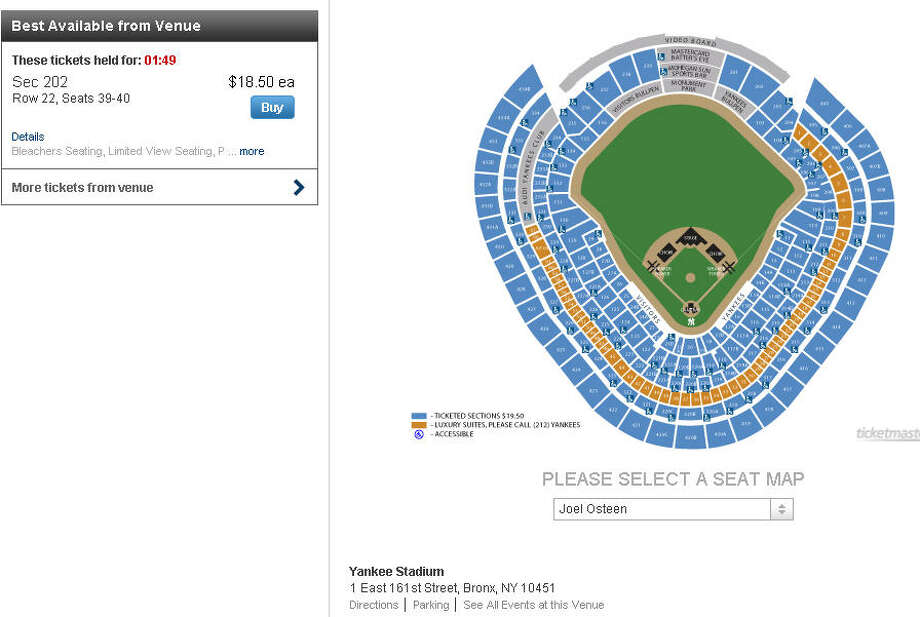A detailed image caption could be:

---

This image, intended for a website where users can purchase tickets, showcases a seating chart for a baseball stadium, presumably Yankee Stadium. The seating chart is color-coded with most sections done in blue, except for an orange strip centrally located and a few sections accented in gray. Due to the low resolution, the text on the chart is not readable. There is a gray text instruction stating, "Please select a seat map," on a white background. 

Central to the image, a drop-down menu indicates "Joel Osteen," suggesting the event is a Joel Osteen gathering at the stadium. The Ticketmaster logo is faintly visible as a watermark and is partially cut off on the right side of the image.

On the left side, a box with a black banner at the top declares "Best Available from Venue." Inside this box, it notes that tickets are held for 1 hour and 49 minutes and specifies seat details as Section 202, Row 22, Seats 39 through 40, priced at $18.50 each. There is a blue "Buy" button with white text below these details, followed by the word "Details." Further text describes the seats and offers a blue hyperlink-like indicator for additional information, likely expanding to show more text upon clicking. Below, black text reads, "More tickets from venue," accompanied by an arrow, indicating interactivity for more options.

---